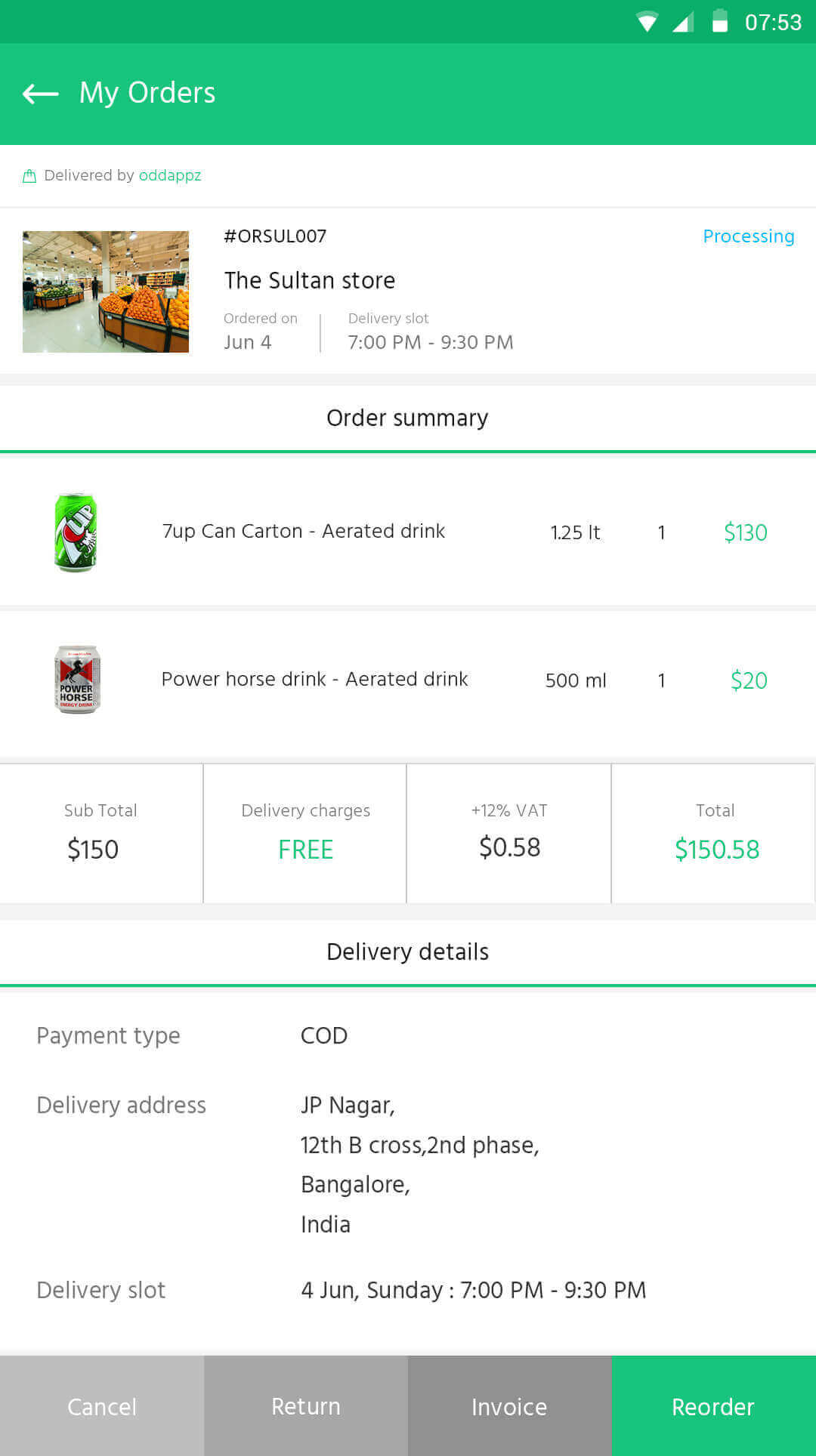This screenshot depicts the "My Orders" menu from an application developed by Odd Apps. The interface features a green header bar with "My Orders" displayed prominently in white text, accompanied by a left-pointing arrow for navigation back to the main menu. Below the header, a note confirms that the service is provided by Odd Apps (spelled O-D-D-A-P-P-Z).

In the main section, there is a thumbnail image showing a supermarket fruit aisle with a shiny marble floor. Various fruits, likely oranges or tangerines, are neatly stacked within the frame. To the right of this image is the order number, labeled as #ORSUL007.

Directly beneath, the vendor identified is the Sultan Store, with the order date noted as June 4th. The delivery window is specified to be between 7:00 PM and 9:30 PM. 

Following this, an order summary is presented. It lists the items purchased, starting with a 1.25-liter can of 7-Up, categorized as an "A-rated" drink, priced at $130, highlighted in green text. The second item is a 500-milliliter Power Horse drink, also classified as "A-rated," costing $20. 

The subtotal for these items is $150. There is no charge for delivery. VAT is calculated at 12%, adding an extra $0.58 to the total. This brings the overall total to $150.58.